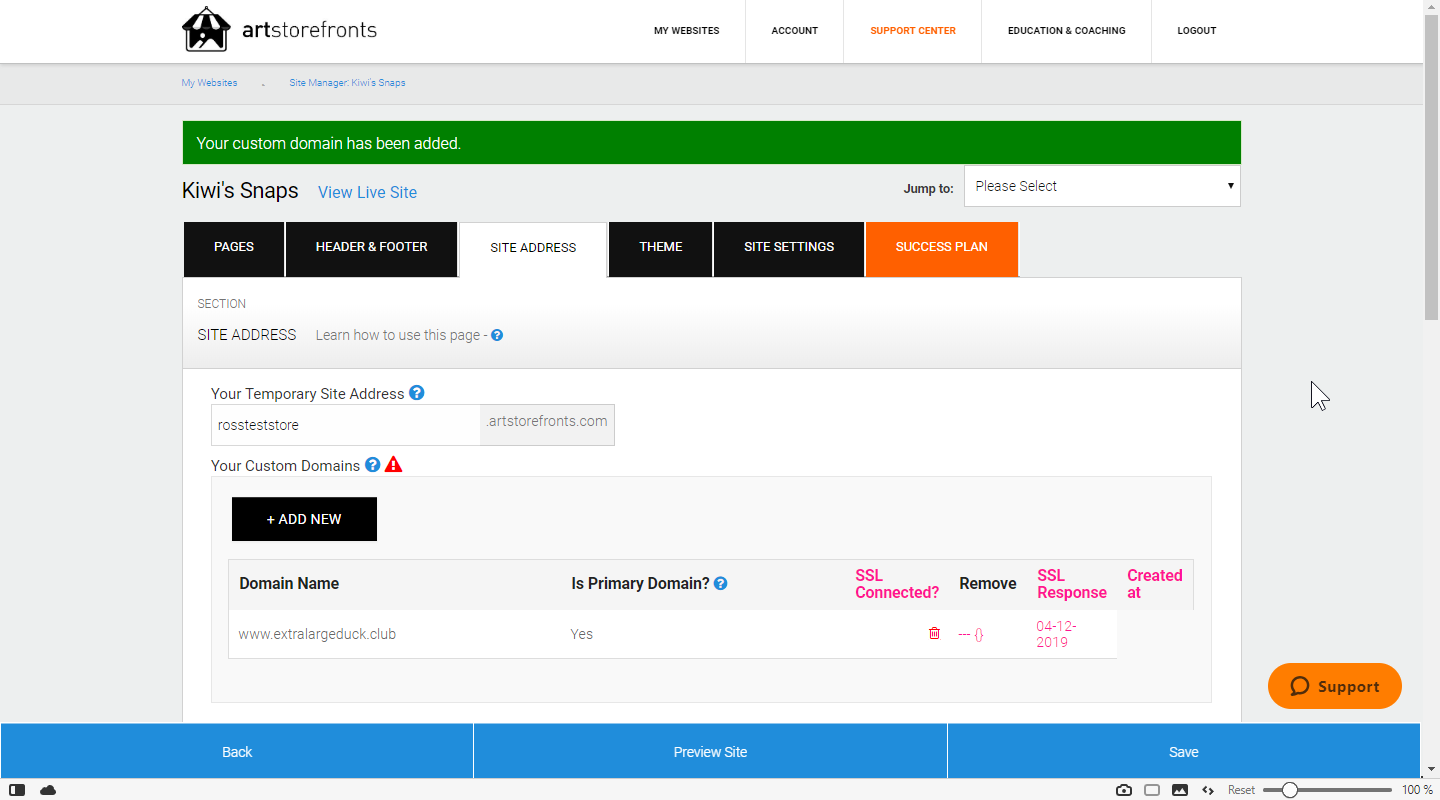### Screenshot Description of Art Storefronts

This image depicts a detailed view of the Art Storefronts management interface. The interface is presented on a gray background and features a distinctive icon of a window with an awning and two mountains, alongside the text "Art Storefronts" in regular font.

To the right, a navigation menu includes the following items separated by vertical gray lines:
- "My Websites" highlighted in blue.
- "Account".
- "Support Center", which is currently selected and marked in orange.
- "Education and Coaching".
- "Logout".

Below the main navigation, the screen displays the section titled "My Websites" in blue. Adjacent to it is the "Site Manager: KiwiSnaps", set against a darker gray bar, while the rest of the content area is light gray. A green horizontal bar spans across the top, stating “Your custom domain has been added” in white text. Beneath this bar, the label "KiwiSnaps" is in black, with a blue "View Live Site" link to the right.

Further right, there’s a "Jump To" dropdown box labeled "Please Select" with a down arrow. Below this are tab options:
- Pages
- Header and Footer
- Site Address (currently selected, colored white)
- Theme
- Site Settings
- Success Plan (highlighted in red/orange)

The section labeled "Site Address" includes:
- A box titled "RossTestStore" with a note about "artstorefronts.com".
- An area labeled "Your Custom Domains" which contains:
  - A red triangle with an exclamation point.
  - A gray box with a black "Add New +" button.
  
Below it lists a custom domain:
- Domain Name: "www.extralargeduck.club"
- Primary Domain marked with a blue circle and question mark to the right indication "Yes".
- Statuses including "SSL Connected" in pink, a red trash can labeled "Remove", and a further note stating "SSL Response 04-12-2019" with its creation date.

To the right of this section is an orange "Support" button. Below the page’s main controls are three buttons in blue:
- Back
- Preview Site
- Save

There is also a status bar featuring symbols indicating battery life at three-quarters full, a cloud, a camera, an empty box, a picture, left and right arrows, a reset button, and a slider set to approximately 20% on a 100-point scale.

This comprehensive view illustrates the Art Storefronts management dashboard in detail.